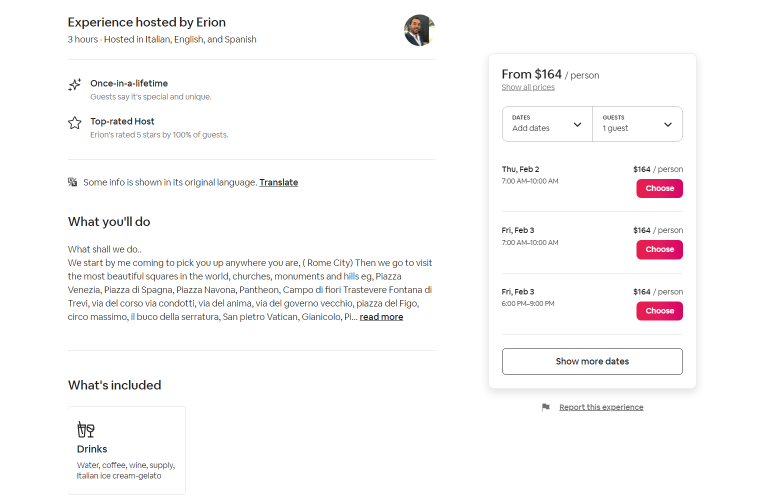This image appears to be a screenshot from the Airbnb app showcasing an exclusive experience hosted by Erion, a highly rated host. At the top of the image, the text states "Experience hosted by Erion," followed by the phonetic spelling "E-R-I-O-N." The description highlights that the duration of the experience is three hours, available in Italian, English, and Spanish. A tagline underneath proclaims it as a "once in a lifetime" experience.

A gray section of text features guest reviews, saying the experience is "special and unique," accompanied by a twinkling four-sided star icon to the left. The text below reads "Top rated host" in black, with an additional note in gray stating, "Erion is rated five stars by 100% of guests," again highlighted with a small star icon next to it.

Further down, some of the information is displayed in its original language, and there's an option to "Translate" shown in black underlined text. The experience description begins with "What you'll do," followed by "What shall we do..." indicating a personalized itinerary. The host, Erion, offers to pick up guests from any location within Rome City, proceeding to visit Rome's most beautiful squares, churches, monuments, hills, and piazzas.

The bottom of the image lists what’s included in the experience, though the specific details are not visible in the provided description.